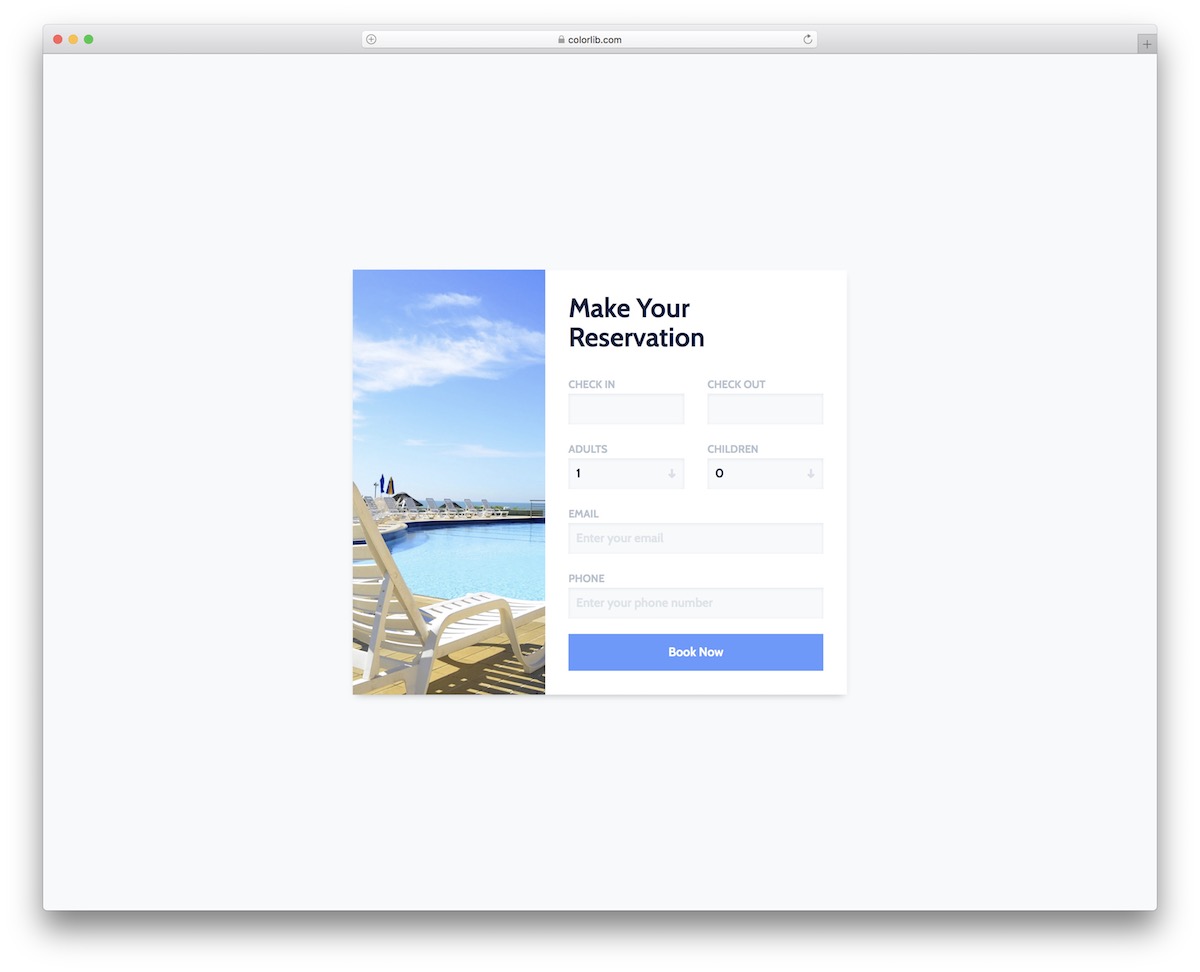A computer screen displays a webpage from colorlib.com, indicated by the browser tab at the top. The main interface of the page is predominantly white, with a central pop-up box that prompts users to "Make Your Reservation." On the left side of this pop-up, there is a stunning image of a swimming pool surrounded by lounge chairs casting shadows on the concrete surface. The pool area is framed by a serene blue sky dotted with fluffy white clouds. On the right side of the reservation box, fields for "Check In" and "Check Out" dates are present. Below these fields, there are sections to specify the number of adults and children for the booking, initially set to 1 adult and 0 children. Additionally, there are input fields labeled "Enter Your Email" and "Enter Your Phone Number," respectively. At the bottom of the pop-up, a prominent blue rectangular button with white text urges visitors to "Book Now."